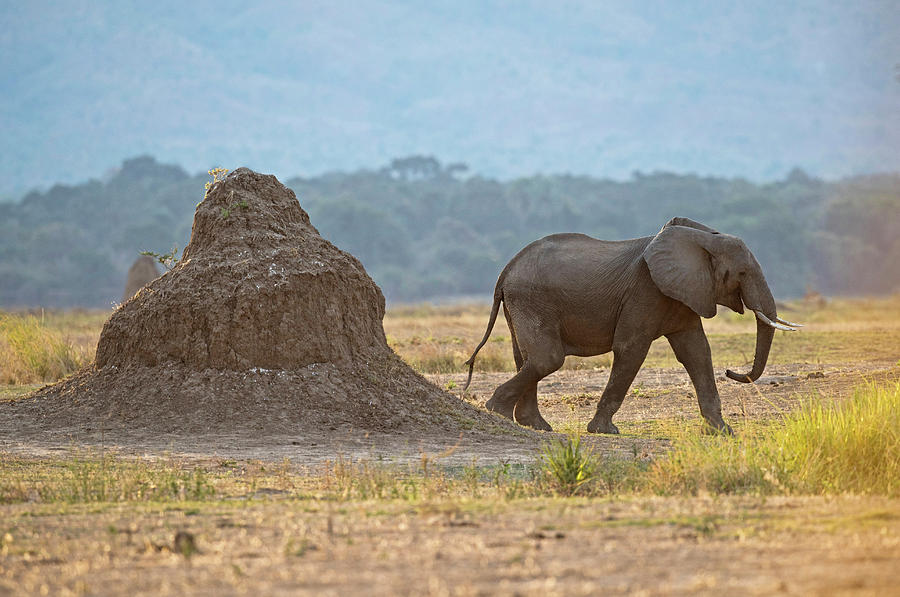This captivating photograph depicts a solitary gray elephant walking across a predominantly barren plain, likely in Africa. The elephant, with both its ivory tusks intact, is positioned on the right side of the image, moving from left to right. Its mouth is slightly open, giving the impression of a gentle smile. The landscape is characterized by a mixture of dry, beige-colored dirt with sporadic patches of yellow grass and weeds.

Dominating the left side of the photograph is a unique rock formation. This intriguing outcrop, taller than the elephant, has a somewhat pagoda-like structure with a dome-on-dome appearance, adding a peculiar yet fascinating element to the scene. Behind this rocky mound, the image reveals a densely forested area extending across the horizon. Above these trees, the sky appears dark, possibly suggesting a cloudy or overcast day, casting a dramatic backdrop against the landscape.

Additional details, such as the glowing orange grass in the sunlight and another similar dirt pile visible in the background, enhance the depth and texture of the image. Overall, the photo captures the serene yet stark beauty of a wilderness scene, with the elephant at its heart, embodying the majestic and enduring spirit of its natural habitat.